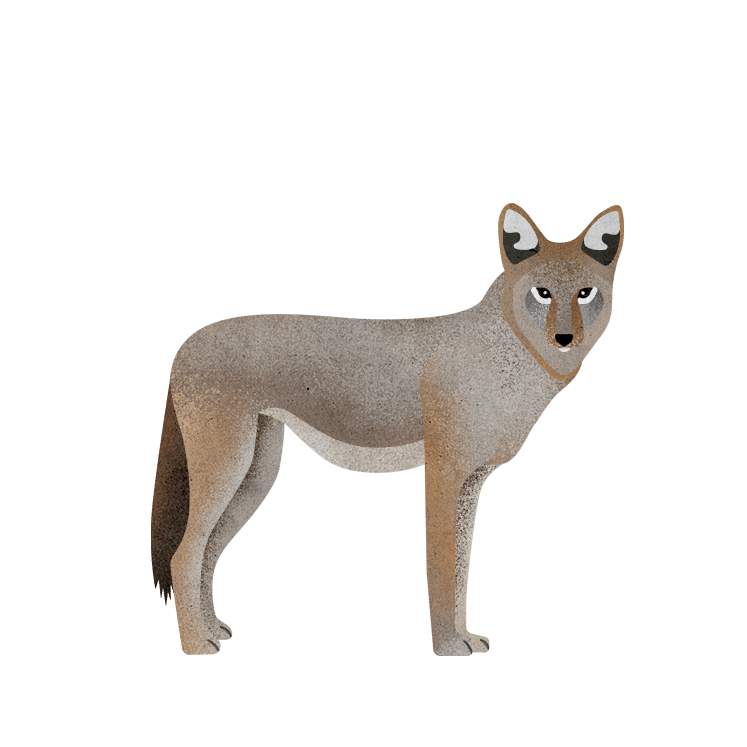This image is a digital artwork depicting a fox in a minimalist style on a solid white background. The fox is shown in profile, facing the right side of the frame, with its head turned toward the viewer. The creature's fur is a mix of gray and brown, with prominent gray splotches beneath its eyes, which are black and white. Its nose is black, and it has a white chin, along with pointed ears that are black and white on the inside. The fox's body shows shading that transitions from gray on the back to brown on the legs and neck, and it features a long, darker brown tail positioned down between its legs. The legs are straight, and the fox stands still, giving it an almost statuesque appearance. The texture of the image suggests a stone-like quality, enhancing the simplicity and elegance of the artwork.